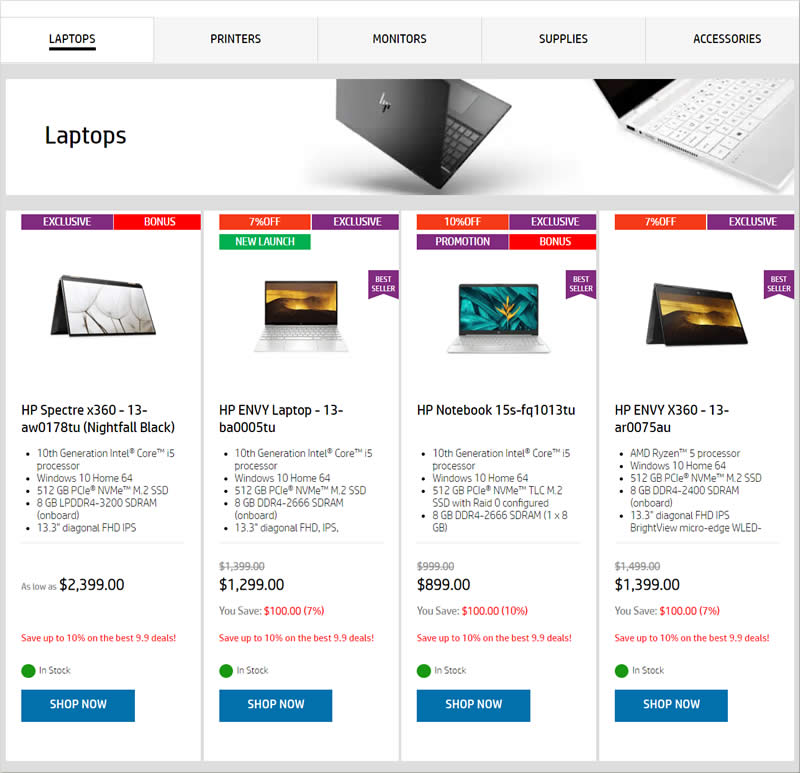Screenshot of a Tech Equipment Display: 

The image showcases a section of a tech equipment webpage, specifically focusing on laptops. At the top, multiple tabs are visible, labeled "Laptops," "Printers," "Monitors," "Supplies," and "Accessories," with the "Laptops" tab currently selected, indicated by bold text. 

The main section features two laptops prominently displayed in a semi-open position, appearing to hover for clear viewing. Below these primary models, four additional laptop options are presented in a grid layout, each with unique selling points highlighted. 

The first option is marketed as "Exclusive," the second offers a "Bonus," the third comes with a "7% off Exclusive" deal, and the fourth highlights another special promotion. Among these, one laptop is shown in an inverted, partially folded position, while the others are arranged normally with front-facing displays. 

All the laptops are HP brand, and there is a noticeable variation in their pricing. The display provides a comprehensive view to help customers compare the different models and promotions available.